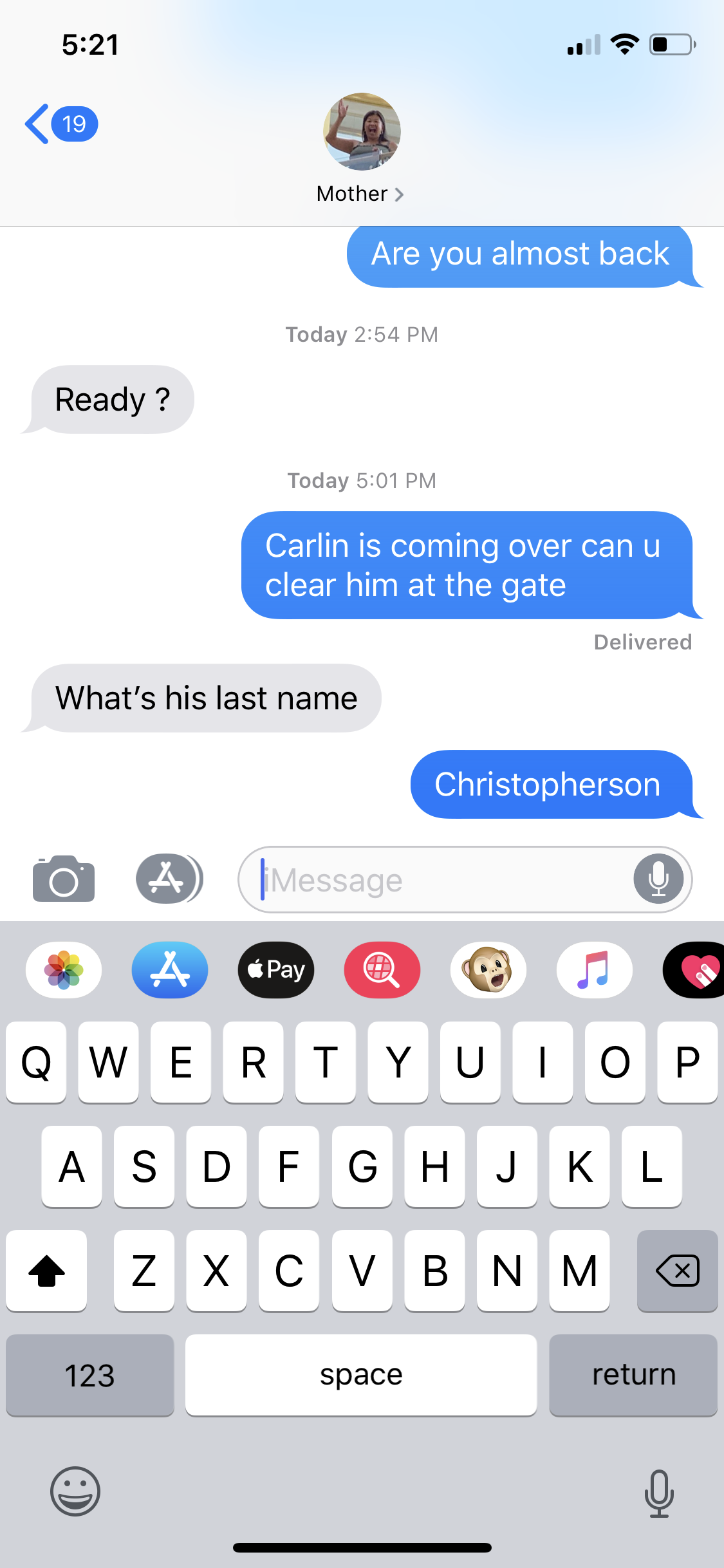The image is a color screenshot of a text message conversation on a cell phone. The top of the screen has a blue gradient band, with a centered circular icon of a woman with short black hair, raising one hand. Below the icon, it reads "Mother" in black text. To the top left of the screen, the time is 5:21, and an arrow with an oval indicates "19,” perhaps referring to new messages. The top right displays a battery icon at less than half charge and two signal bars. 

The text conversation itself spans the middle section of the image, featuring blue and gray speech bubbles. The first message on the top right in a blue bubble reads, "Are you almost back?" at 2:54 PM today. A gray bubble on the left follows, asking, "Ready?" A subsequent blue bubble on the right at 5:01 PM today reads, "Carlin is coming over, can you clear him at the gate?" This message is noted as "Delivered." The conversation continues with a gray bubble on the left asking, "What is his last name?" and concludes with a blue bubble on the right stating, "Christofferson."

Below the conversation, the phone's keyboard is visible, displaying QWERTYUIOP, ASDFGHJKL, and ZXCVBNM, with additional keys for punctuation, space, and return. Icons for emojis and the microphone are at the bottom left and right, respectively.